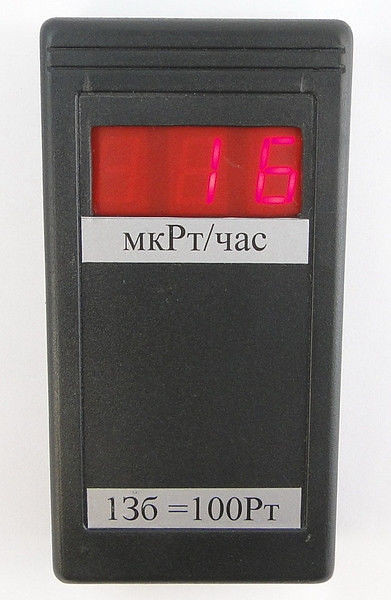This indoor, close-up photograph features a dark gray, rectangular plastic device with smooth corners, set against a white background. The focal point is a red rectangular LED display at the upper half of the device, currently showing the numbers "16" in a pinkish-red hue. Below the LED display, a white rectangular label reads "MK PT/yac," with "MK" and "PT" in uppercase and "yac" in lowercase. Further below, another white rectangular label at the bottom of the device states "136=100P" with a smaller "T" next to it. The upper part of the device's casing has vertical ridges molded into it, adding a textured element, while the lower part appears smooth. The overall condition of the device is excellent, with no visible nicks, mars, or dirt. No additional text or labels are present outside of those described, and there are no distinguishing features or items in the background, making the image solely focused on the device itself. This item may potentially be a thermostat or a similar electronic display apparatus.